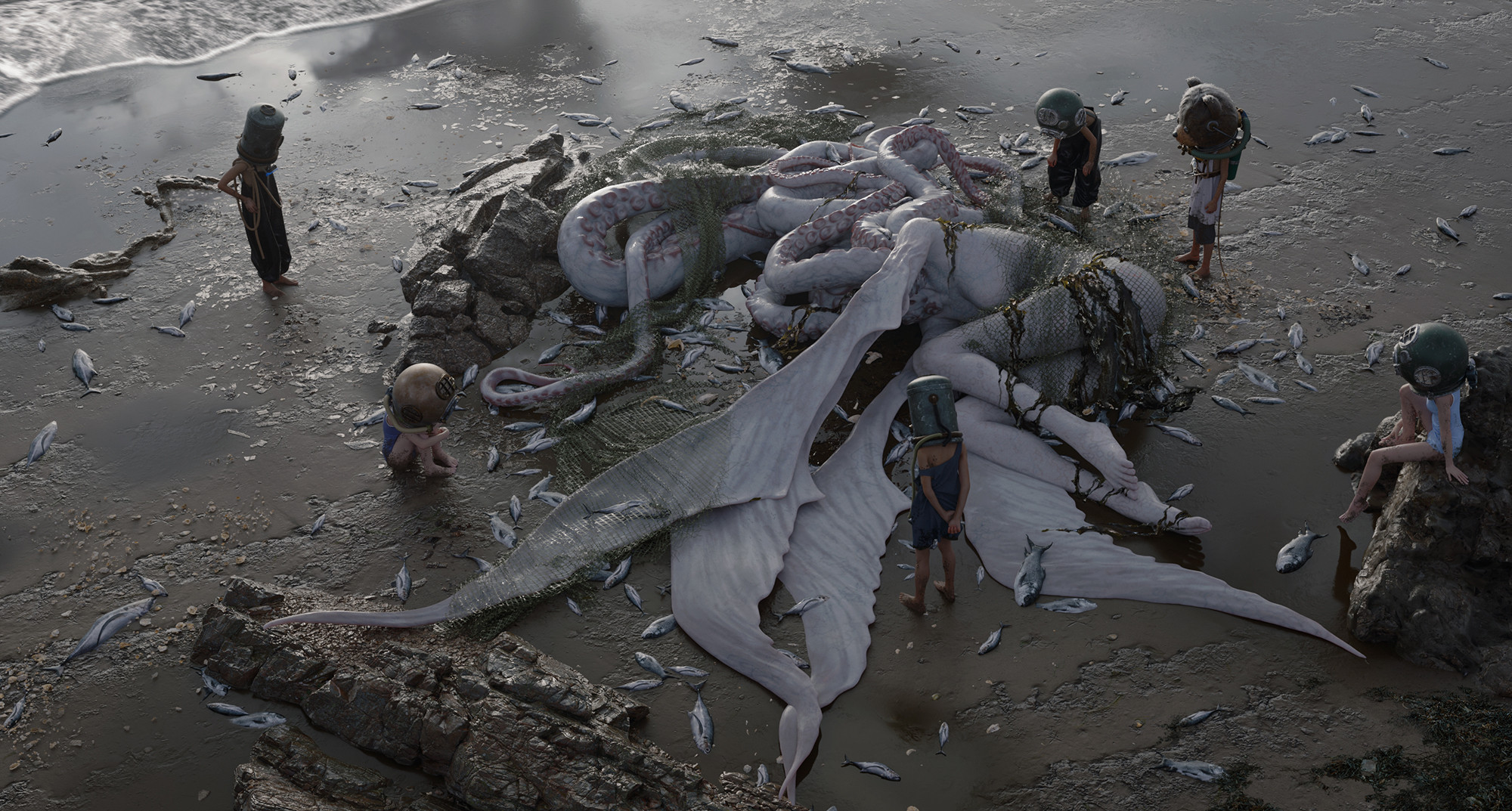The image depicts a surreal scene set by the sea. At the center, a bizarre creature combines human and marine features: a humanoid body with human legs and hands that end in wings. Its head is an octopus, adorned with tentacles. The creature, pale in color, appears to have been washed ashore. Surrounding it, several fish are scattered, also washed up by the sea, along with patches of seaweed draped over the creature.

In addition to the marine elements, six human figures encircle the creature. These individuals are dressed in swimsuits, but notably, their heads are obscured by buckets. The overall aesthetic of the image suggests it is not a genuine photograph but rather an artistic creation, possibly a still from a movie or a digital artwork.